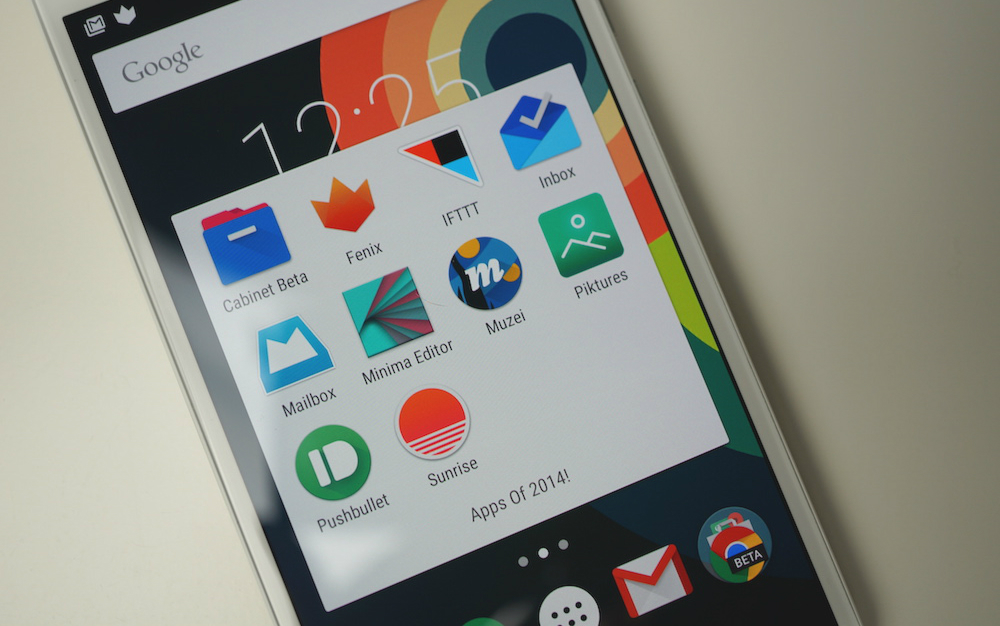The image showcases a smartphone device with light grey, almost silver edges set against a cream white background. The device's screen displays a Google search bar at the top alongside a Gmail icon. Below these, multiple icons for various applications are arranged, each with distinct designs and color schemes. 

Prominent app icons include:
- "Pictures" with a green and white icon featuring an image symbol.
- "Muse" with a white, blue, and orange icon.
- "Minimoid Data" with a green and red icon.
- "Mailbox" with a blue and white icon.
- "Push Purchases" with a green and white icon.
- "Sunrise" with a red and white icon.
- "Carbonate Beta" with a blue and red icon.
- "Phoenix" with an orange icon.
- "IFTTT" with a black, red, and blue icon.
- "Inbox" with a blue and grey icon.

The time displayed on the smartphone is 12:25. At the bottom of the screen, additional icons, including Gmail and Beta Chrome, are visible. The text "Apps of 2014" is displayed, indicating a collection of noteworthy applications from that year, such as Carbonate Beta, Phoenix, IFTTT, Inbox, Mailbox, Minimoid Data, Muse, Pictures, Push Purchases, and Sunrise.

The background of the central tab is grey, while the wallpaper spans a black canvas accented with streaks of red, orange, yellow, green, and dark blue tones.